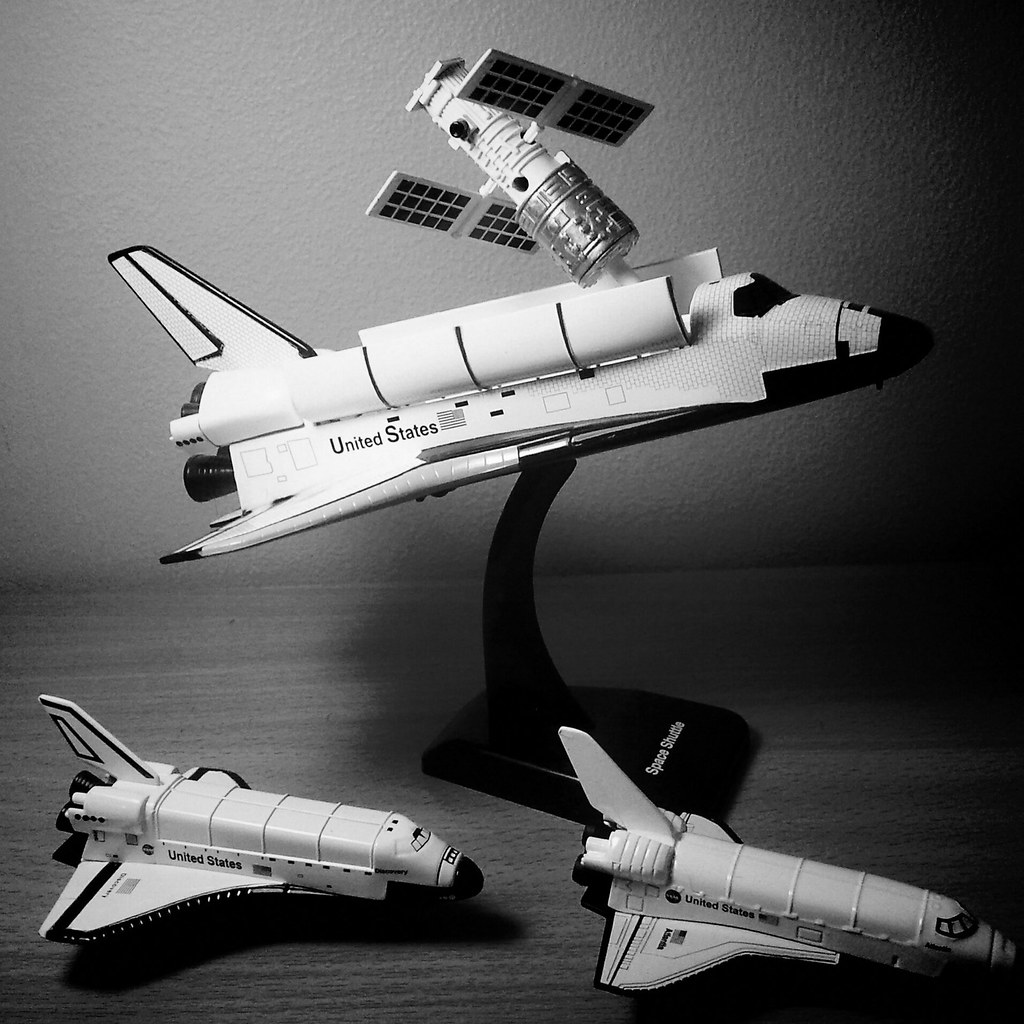This black and white photograph captures a detailed display of three model spacecraft on a textured light-colored wall background. The models are positioned on a darker wood grain desk that extends across the foreground. The centerpiece of the image is a prominent, long model space shuttle mounted on a black trapezoidal stand inscribed with the text "Space Station." This large shuttle, predominantly white with a black pointed nose, bears the inscription "United States" alongside an American flag. Attached to the top of this shuttle is a white and metallic cylindrical mechanism, likely a satellite, with two checkered rectangular panels extending from its sides.

Below and in front of the large shuttle are two smaller, almost identical, model shuttles. These smaller shuttles mirror the design of the larger one, complete with white bodies, black pointed noses, and black rocket nozzles at their rear. Each of these smaller models also features the "United States" text on their sides. The overall composition creates a visually striking and detailed exhibit of space exploration models, set against a contrasting backdrop that highlights the intricate designs of the spacecraft.